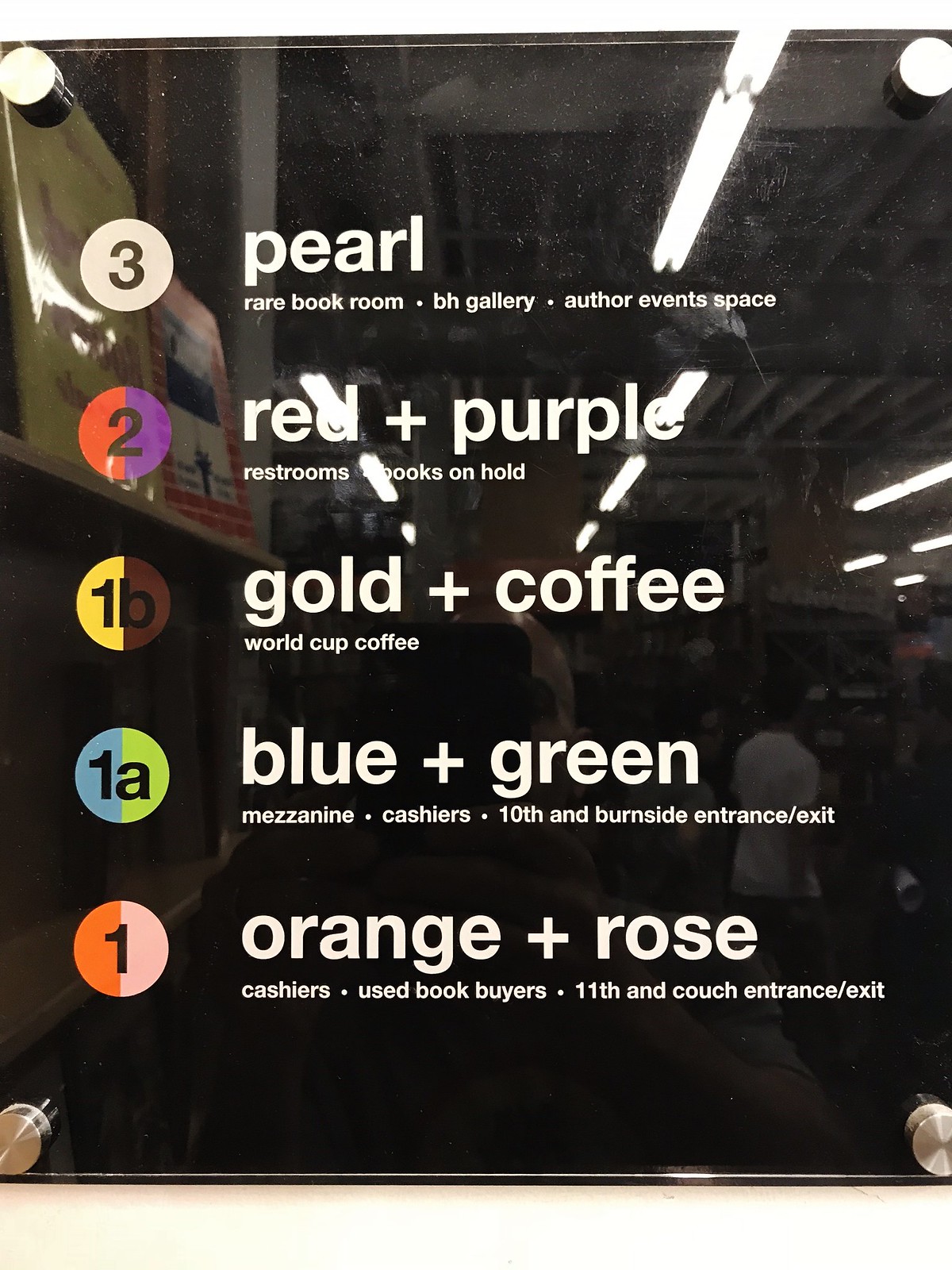In this visually captivating image, the central element appears to be a chart on a sleek, glossy black background. Each corner of the chart is accentuated with what looks like silver nails, adding a touch of vintage charm. 

Prominently featured at the top is a white circle with a bold black number "3," and under it, the text "Pearl, Rare Book Room, Ben Gallery, Author Event Space," all written in crisp white lettering. 

Beneath this, there is a striking half-red, half-purple circle with a black number "2" inside. Surrounding this circle, the text reads "Red and Purple: Restrooms, Books on Hold," indicating those key locations.

Further below, a half-gold circle with a black number "1" directs attention to “Golden Coffee, World Cup Coffee,” suggesting these are notable spots to find a caffeine fix.

Adding to the array is a half-blue and half-green section bearing the label "1A." This part of the chart denotes areas labeled "Blue and Green: Mezzanine Cashiers, 10th and Burnside Entrance/Exit."

Finally, the lower portion of the image features a half-orange half-pink segment labeled with the text "Orange and Rose: Cashiers, Used Book Buyers, 11th and Couch Entrance,” rounding off the guide to various significant areas.

Each color-coded section provides an organized and visually appealing representation of the various locations within the described space.